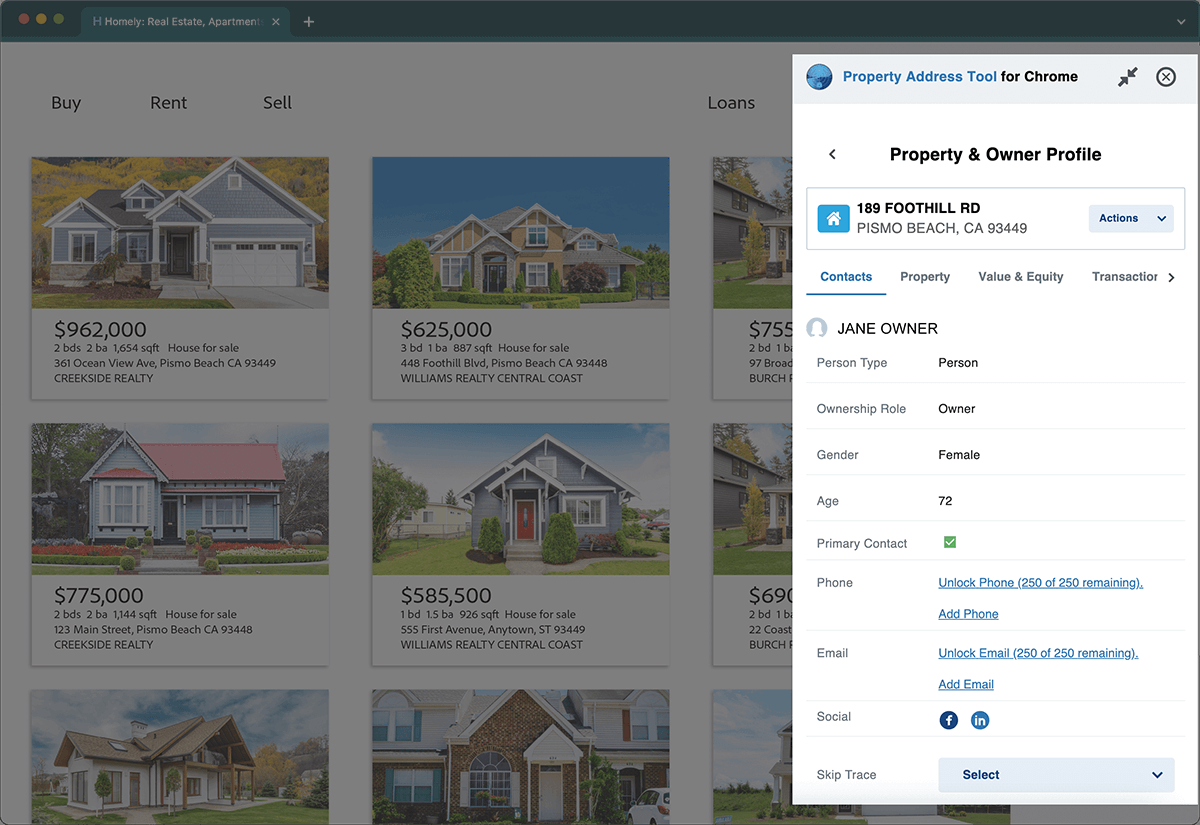This image depicts a screenshot of a real estate platform named "Homely: Real Estate, Apartments," partially visible at the top of the screen. The interface has clear sections for 'Buy,' 'Rent,' and 'Sell,' accessible from the main menu. The background is filled with numerous property listings that range in price from $185,500 to $962,000, all located in Pismo Beach, California.

On the right side of the screen, the user has selected a specific property and owner profile. The address of the property is 189 Foothill Road, Pismo Beach, California. The profile includes detailed information such as the owner's name, Jane, who is a 72-year-old female and the primary contact for this property. Additional details include her phone number, email address, social media links, and their website. The profile also provides information on the property's value, equity, and past transactions. The overall layout offers a comprehensive view of the real estate market in Pismo Beach, CA, along with detailed profiles for specific properties and their owners.